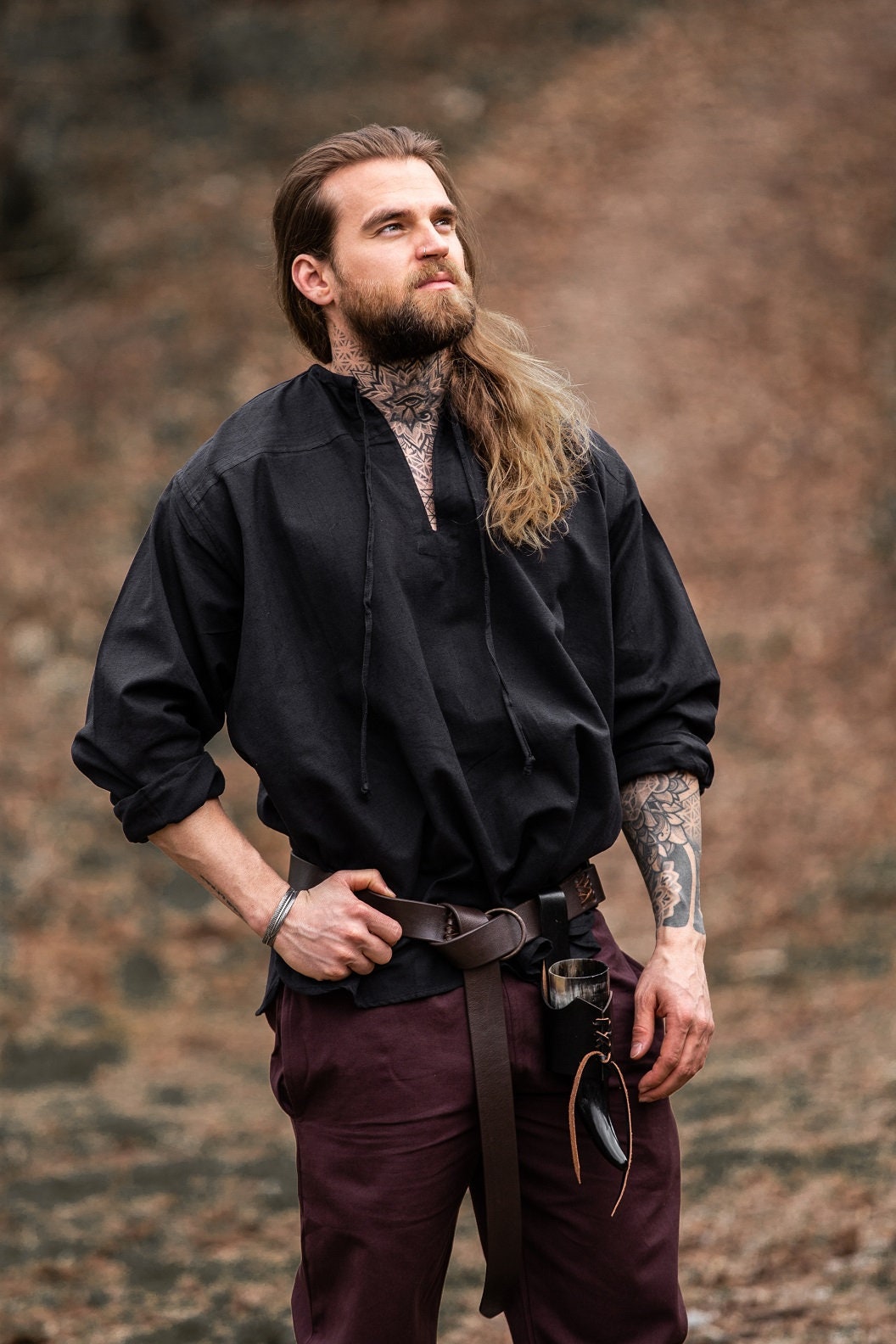The photograph captures a man standing in a wooded area during fall, evidenced by the yellow and brown leaves scattered across the ground. The background is blurry, emphasizing the man who is looking up towards the sky. He has long brown hair that drapes over his left shoulder and a brown beard. A star tattoo is visible on his neck. The man is dressed in a black v-neck pullover shirt that has ties for adjusting the neckline and maroon pants. A leather belt is looped around his waist, tied in a knot, from which a horn and a knife in a holder, with a black handle, hang. His left arm sports a flower tattoo while his right wrist is adorned with a metal bracelet. He holds his left hand on his hip and lets his right arm hang down. The overall attire and accessories suggest a style reminiscent of medieval or Renaissance fair clothing.